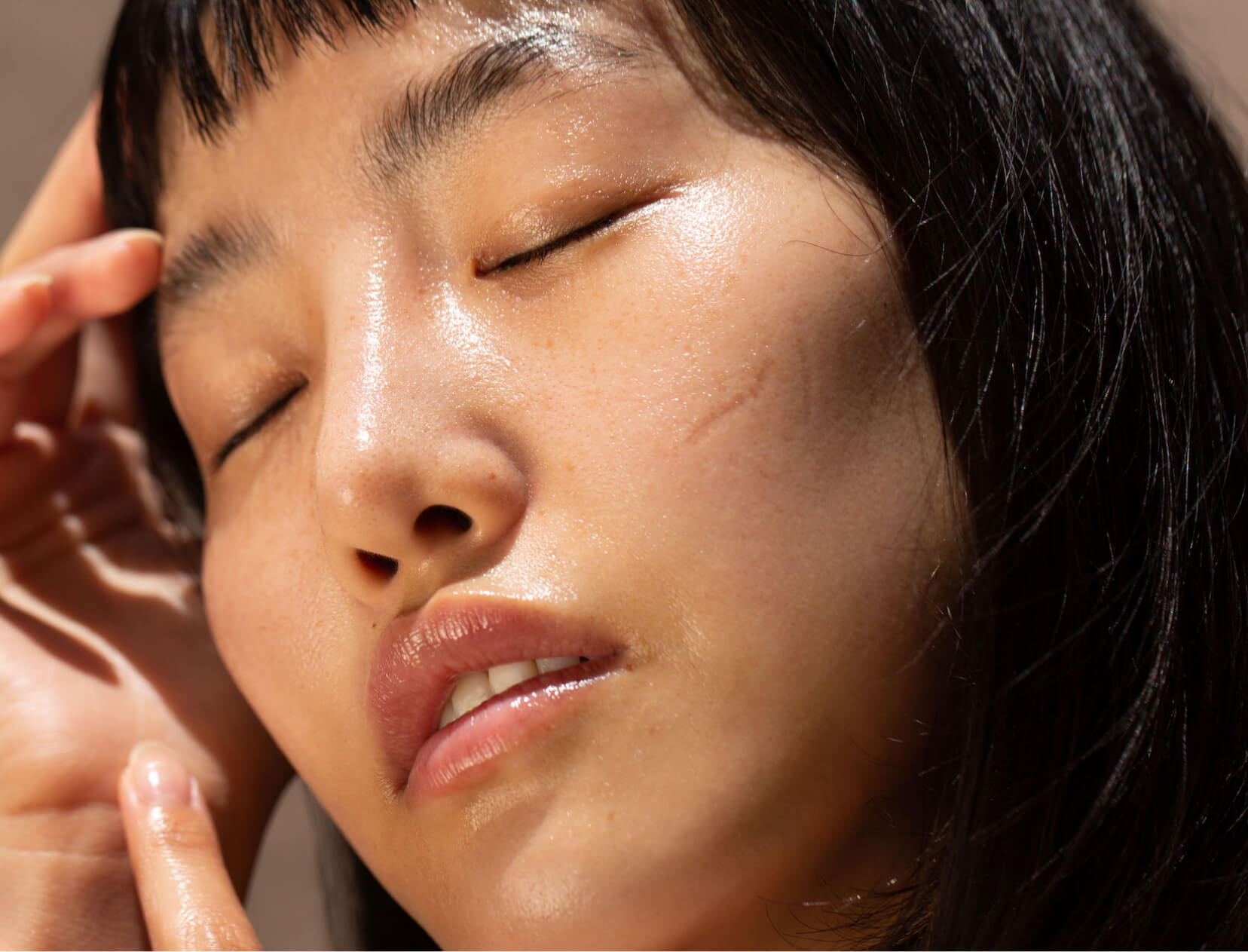This image is an extremely close-up shot of the face of an Asian woman with short black bangs and medium-length black hair, which falls around her face in a bob style. Her eyes are closed, and she appears to be either sleeping or in a state of nervous contemplation. Her head rests on one hand, which supports her tilted face, while her other hand touches the palm of the supporting hand. She has fair skin and a small, horizontal scar about an inch long below her left eye. Her eyebrows are dark and sparse, and her short eyelashes frame her closed eyes. Her mouth is slightly open, revealing the bottom section of her top teeth. Her lips are full and pink, possibly with a hint of lip gloss. The absence of makeup emphasizes her natural appearance. Although one woman's nails are described as unmanicured, they are also noted to be long and nicely manicured, extending just past the ends of her fingertips. The lighting casts a slight shine on her face, enhancing the texture of her skin.